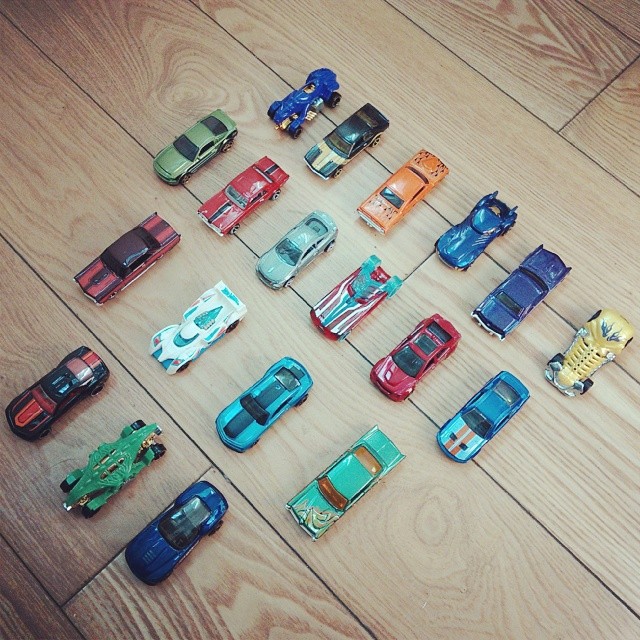This photograph captures a top-down view of a light brown tile floor with black grout lines, displaying a meticulously arranged collection of 19 small matchbox cars. Organized into four rows of progressively increasing quantity—starting with three cars in the first row, followed by four cars in the next, and six cars each in the subsequent two rows—each car is symmetrically spaced, much like dominoes. The colorful variety includes multiple shades of blue, from light to dark, with notable appearances of red, green, yellow, and a single orange car. Specific cars stand out, such as a black one featuring a yellow "T" on its hood and a striped red and blue vehicle, possibly resembling a racing car. The positioning and careful spacing suggest a child's playful arrangement, with the cars' compact designs and bright hues evoking a sense of organized, whimsical fun.